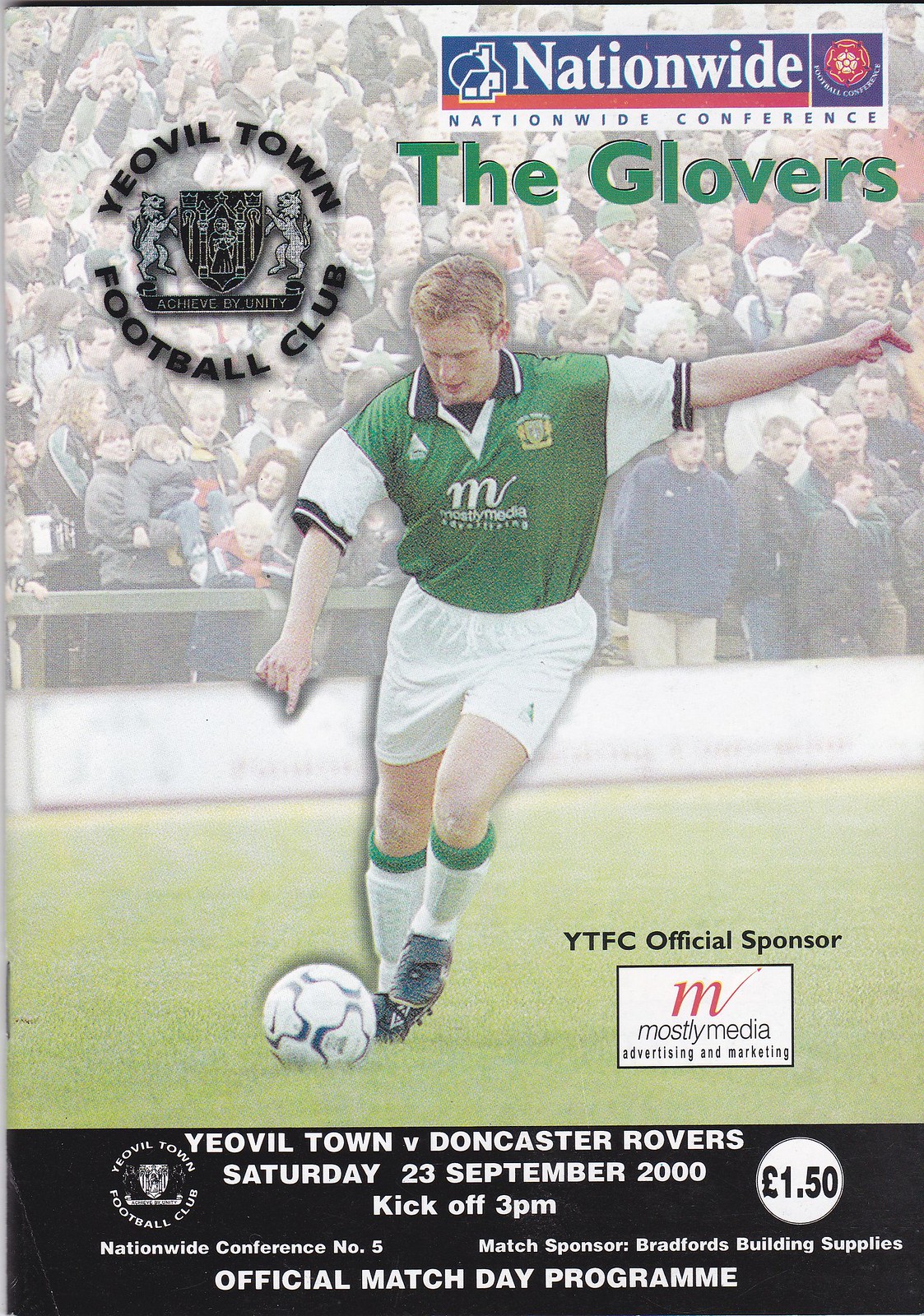This detailed caption brings together the repeated and emphasized elements from each description:

---

The front cover of the official match day program for Yeovil Town Football Club, known as The Glovers, features a dynamic image of a player in mid-kick. The player dons a green and white jersey with a blue collar and blue sleeve accents, white shorts, and prominently a white 'M' logo on the center of his jersey. Behind the player, a large crowd of spectators is visible. 

In the upper right corner, there is a blue box with white letters that read "Nationwide," followed by "Nationwide Conference," underlined by a red line, and accompanied by their symbol in a square. The top also features the text "Vivo Town Football Club" (likely referring to Yeovil Town FC) along with a suit of arms logo.

Adjacent to the player's feet on the right side is a white box containing a red 'M' and the text "Mostly Media, Advertising, and Marketing," with "YTFC Official Sponsor" positioned above it.

The bottom of the cover has a large black border with white text detailing the match information: "Yeovil Town vs. Doncaster Rovers, Saturday, 23rd September 2000, Kickoff at 3 p.m., Nationwide Conference No. 5, Match Sponsor Bradford's Building Supplies," and concluding with "Official Match Day Program." Additionally, within a white circle with black lettering, the price "£1.50" is specified.